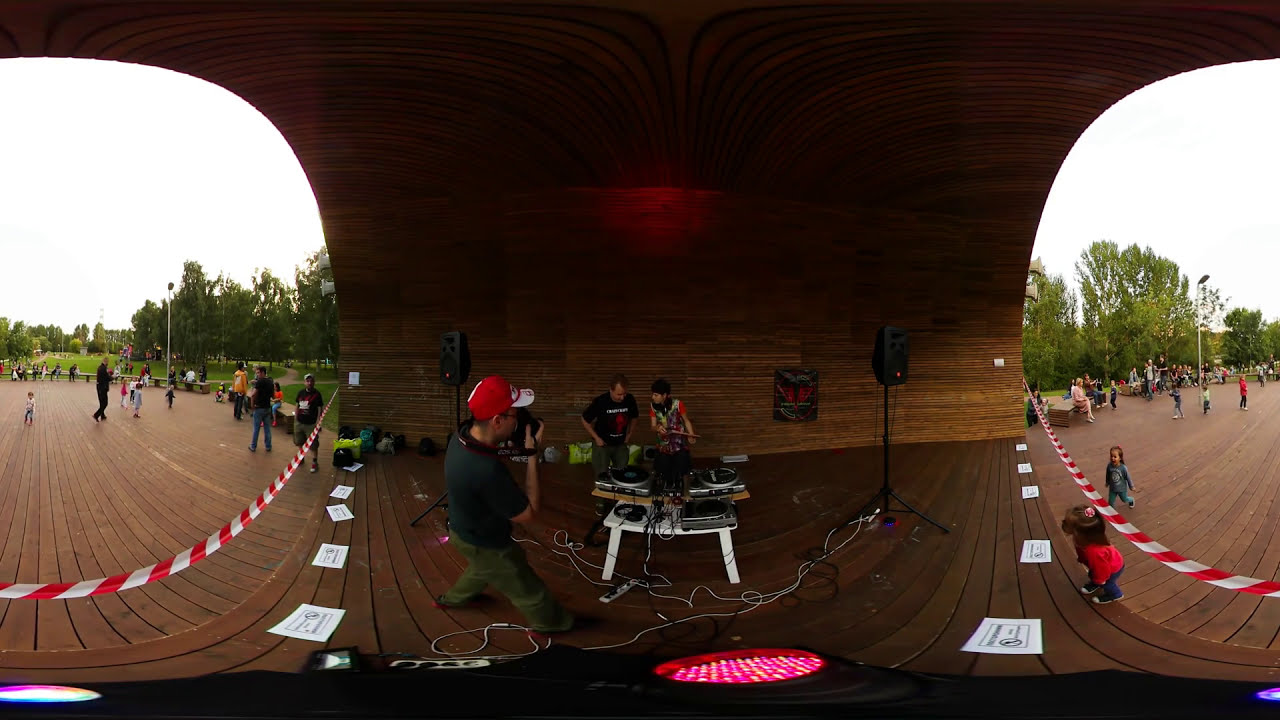This color photograph captures an intriguing outdoor scene, predominantly showcasing a covered area that resembles a pavilion, possibly under a tunnel or highway underpass, where people appear to be setting up for an event - likely a musical or radio station performance. The central focus is a white table laden with electronic equipment, including turntables and audio systems, suggesting substantial preparation for the upcoming event. Behind the table, two individuals are engaged in the setup: a man wearing a black t-shirt with white writing, and beside him, a woman in a tan jacket leaning forward, inspecting the devices. 

In the foreground stands a man in olive green pants, a black t-shirt, and a red baseball cap, holding a camera to document the scene. On either side of the arched structure, which is lined with wooden pathways and adorned with cautionary red and white striped tape, a park-like setting unfolds, featuring red brick walkways. Visible on the left, near a red and white striped walkway, a man plays with children against a backdrop of a tree-lined horizon meeting a cloudy, white sky. Similarly, on the right, children and adults gather, with some children appearing curious about the preparations under the overpass.

The overall ambiance suggests a vibrant community space, merging indoor and outdoor elements, with people milling about, children playing, and the anticipatory buzz of a public event in an extensive outdoor park.